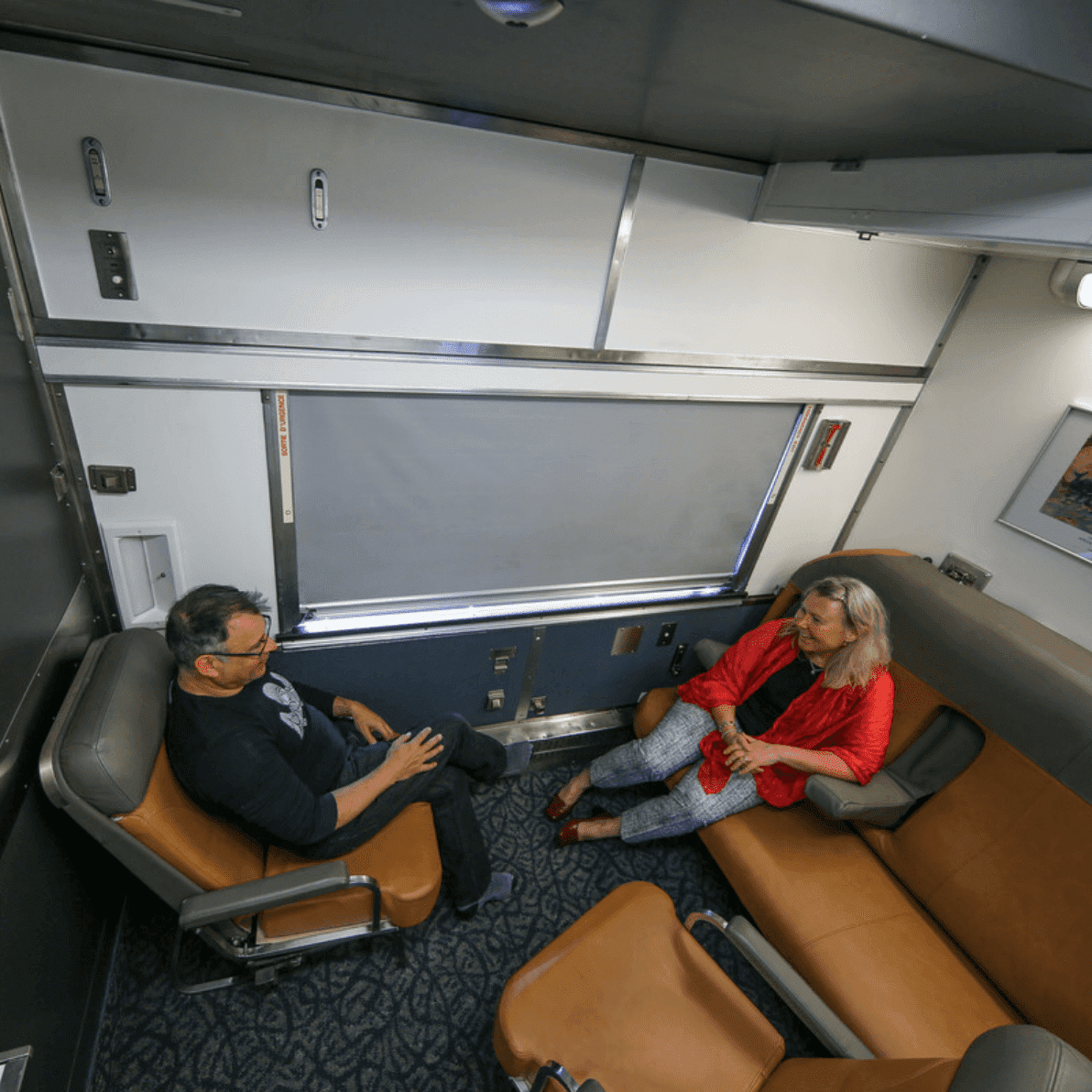This image captures an intimate moment between a man and a woman seated in what seems to be a private train compartment, likely within a mobile home or RV. Taken from an upward angle, the photo shows them sitting across from each other on brown and gray leather seating. The man's chair is on the left and the woman's, resembling a small couch, is on the right. An empty chair, identical in color, sits between them. The man, who has glasses and grayish-brown hair, wears a black shirt with a white character, black jeans, and socks. His hands are resting on his crossed legs, and he is smiling. The woman, appearing to be in her late 40s or 50s, has graying hair, and is laughing. She is dressed in a red cardigan over a black shirt, complemented by gray pants and red shoes. Her arm rests on the armrest. The compartment features a distinctive gray and dark gray patterned carpet, white paneled walls with silver trim, and a large rectangular window covered by a gray shade. Behind the woman, a framed picture hangs on the wall. Soft lighting illuminates their happy exchange, suggesting a moment of pleasant conversation during their journey.